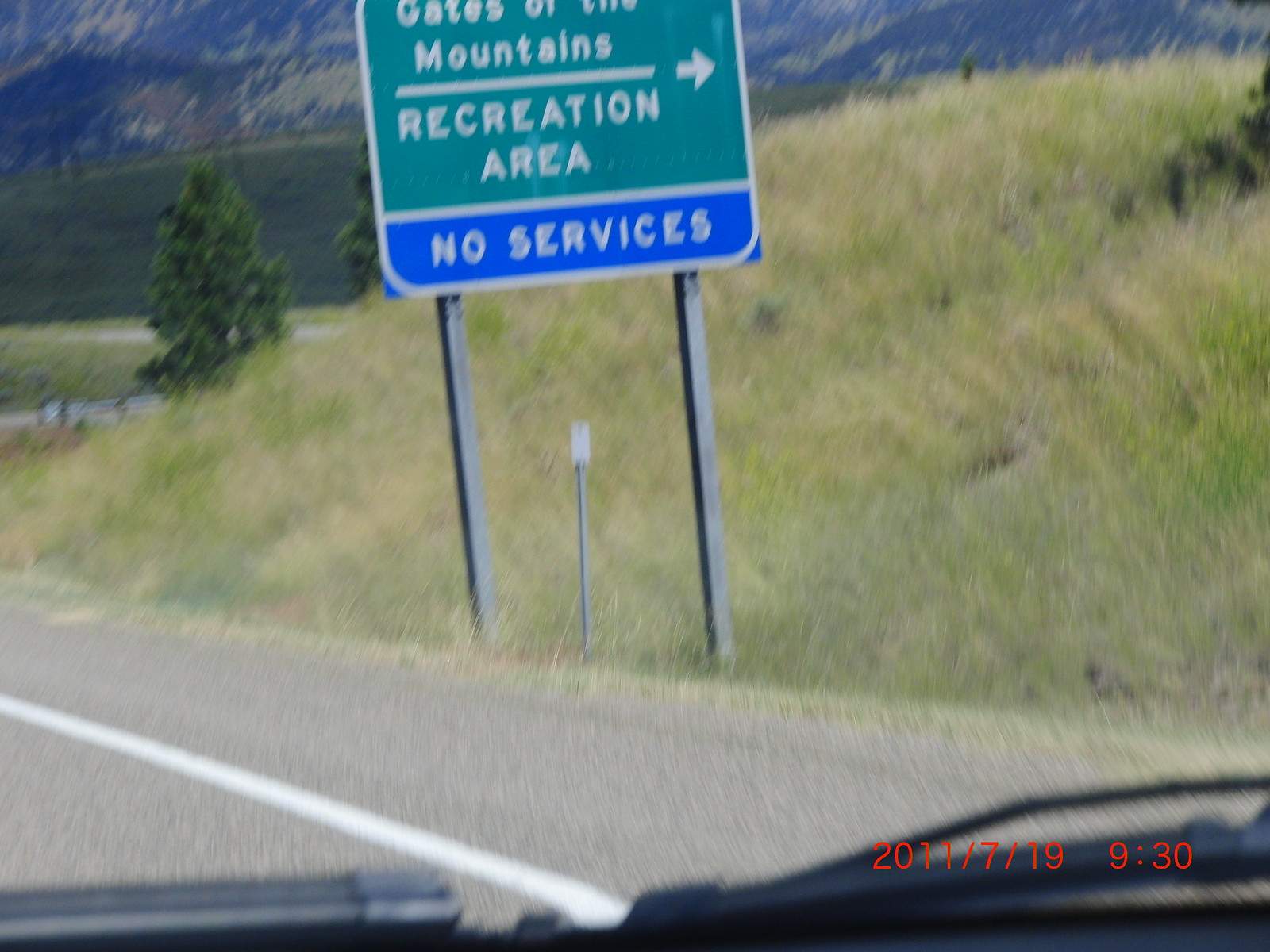The image captures the view from inside a car, looking out through the front windshield onto a scenic area. Dominating the center of the scene is a roadside sign with a green background and a small blue border at the bottom. The sign, square in shape, reads "Gates of the Mountains Recreation Area" with an arrow pointing to the right, and below in the blue border, the words "No Services" are clearly displayed. The setting around the sign features rolling grassy hills and majestic mountains in the distance. The road in front of the car appears to be a standard traffic road, colored light green, with a white line running from the bottom center of the image to the bottom left. Additionally, the bottom right corner reveals a part of the car's windshield wipers, indicating the vantage point of the viewer inside the vehicle.